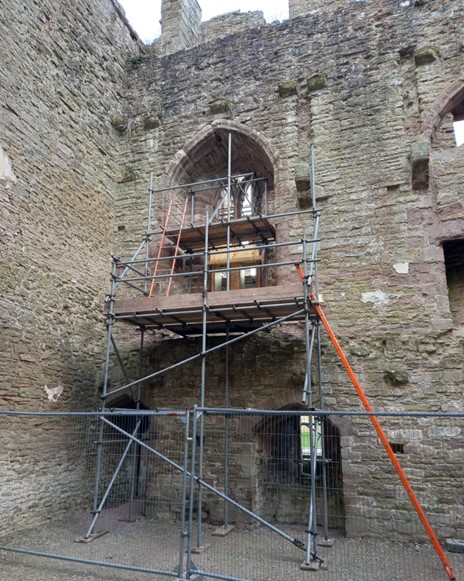The image features a very old and decrepit building primarily constructed out of gray and brown stone, with evidence of black mildew staining towards the top. The lower sections of the building display remnants of deteriorating brick, and the entire structure exhibits significant wear and dirt. The building's façade includes an open entryway at the bottom and a few window openings scattered throughout. In the middle of the image, and extending towards the top, a network of silver metal scaffolding stands prominently in front of the structure. This scaffolding includes a series of platforms, with an orange ladder positioned against it, climbing upwards to reach additional levels. A new iron fence runs along the bottom front of the building, likely to restrict access and ensure safety around the construction site. Behind the fence, to the right, another orange ladder ascends further, connecting to a platform with another ladder on top of it. Amidst the scaffolding, there is a brown door subtly visible behind one of the ladders, emphasizing the ongoing work and structural complexity. The bottom of the image reveals a dirt ground, devoid of any significant features.